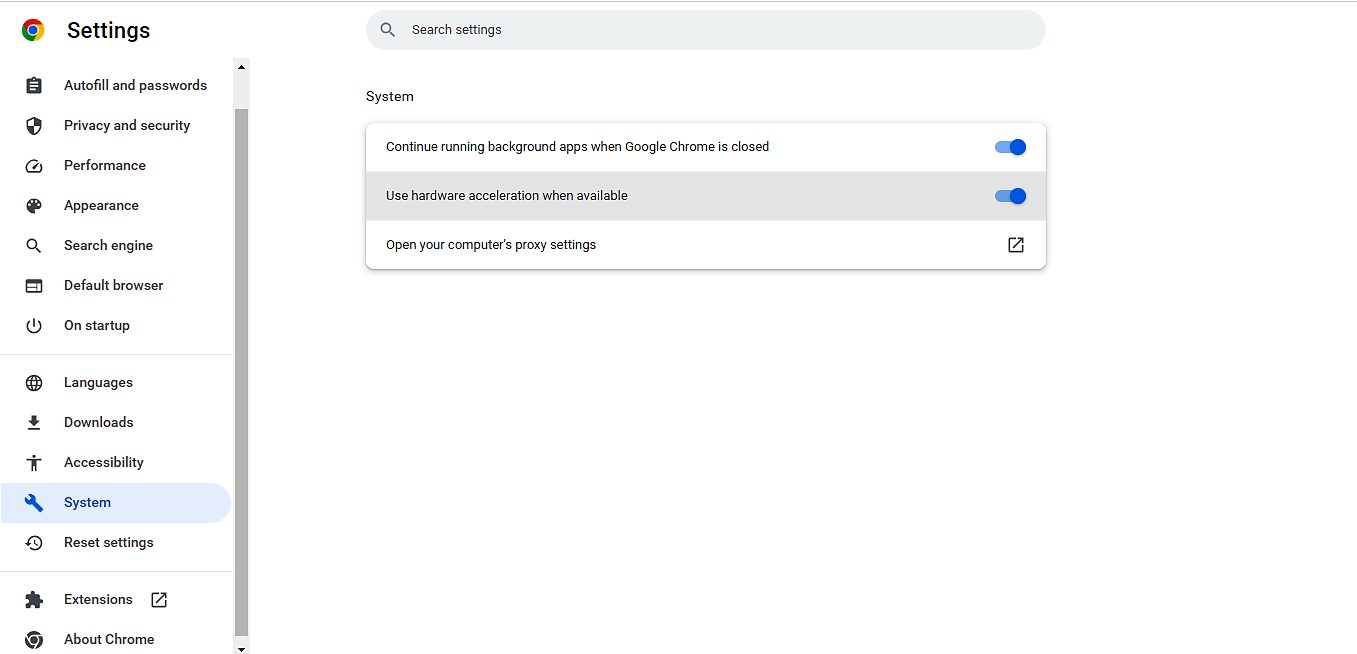This image showcases a Google Chrome settings page, meticulously detailed and structured for user customization and management. On the left side of the page, a prominent Google icon resides, accompanied by the word "Settings" immediately to its right.

The settings are organized into a vertical list of categories. First on the list is "Autofill and Passwords," followed sequentially by "Privacy and Security," "Performance," "Appearance," "Search Engine," "Default Browser," and "On Startup." A delicate gray divider line segments the primary settings from other options. Below this divider, the list continues with "Languages," "Downloads," "Accessibility," "System," which is the currently selected section and highlighted in blue, "Reset Settings," "Extensions," and "About Chrome."

Moving to the main body of the page, a search box designed for locating specific settings is positioned at the top. Directly beneath it is the "System" category content. This section comprises three distinct options with corresponding toggle buttons: "Continue running background apps when Google Chrome is closed," which is currently activated, "Use hardware acceleration when available," also activated and highlighted, and "Open your computer's proxy settings."

This comprehensive visual and textual representation of the settings page provides a clear, full-featured view of the system configurations and customization options available to users within Google Chrome.